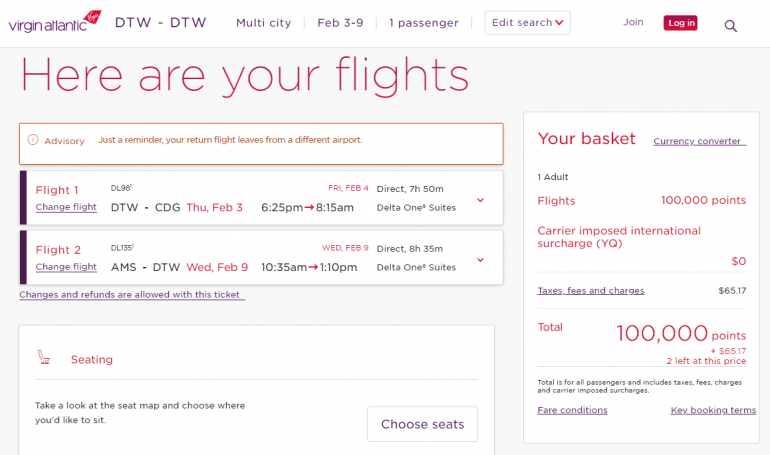The image features a light purple background with a detailed breakdown of flight information for a Virgin Atlantic booking. 

At the top, the text "Virgin Atlantic" appears in purple with a small pink icon to its right. The details of the booking are shown as "DTW to CDG, multi-city, February 3rd through 9th, one passenger," along with an "edit search" box that includes a red down arrow. Following this, there's a command for users to "join," and a bright pink box labeled "log in," accompanied by a magnifying glass icon.

Below this, the text "Here are your flights" stands out in bright pink on the light purple background. There is also a pink advisory box featuring a clock icon with a message: "Just a reminder, your return flight leaves from a different airport."

The flight details are presented in separate boxes with a dark purple line on the left side:

- **Flight One:**
    - BL 96 DTW to CDG
    - Thursday, February 3rd from 6:25 AM to 8:15 AM (next day, direct, 7 hours 50 minutes)
    - Delta One Suites
    - "Change flight" option available in purple, underlined
    - Pink down arrow icon

- **Flight Two:**
    - DL 130 AMS to DTW
    - Wednesday, February 9th from 10:35 AM to 1:10 PM (direct, 8 hours 35 minutes)
    - Delta One Suites
    - "Change flight" option available in purple, underlined
    - Pink down arrow icon

Highlighted in pink, the phrase "Changes and refunds are allowed with this ticket" is underlined for emphasis.

Towards the bottom, two additional boxes offer more options:

- The first box, titled "Seating" in pink, showcases an icon of a seat. It invites users to "take a look at the seat map and choose where you'd like to sit," along with a "choose seats" button.

- The second box, labeled "Your Basket" in pink, contains a "currency converter" option in purple, underlined. It breaks down the flight costs for one adult: 
    - Flights: 100,000 points
    - Carrier-imposed international surcharge (YQ): $0
    - Taxes, fees, and charges: $65.17
    - Total: 100,000 points plus $65.17
    - "Two left at this price" note, emphasizing the urgency
    - "Total is for all passengers and includes taxes, fees, charges, and carrier-imposed surcharges"
    
Finally, the options "fare conditions" and "key booking terms" are displayed in purple and underlined, providing additional information.